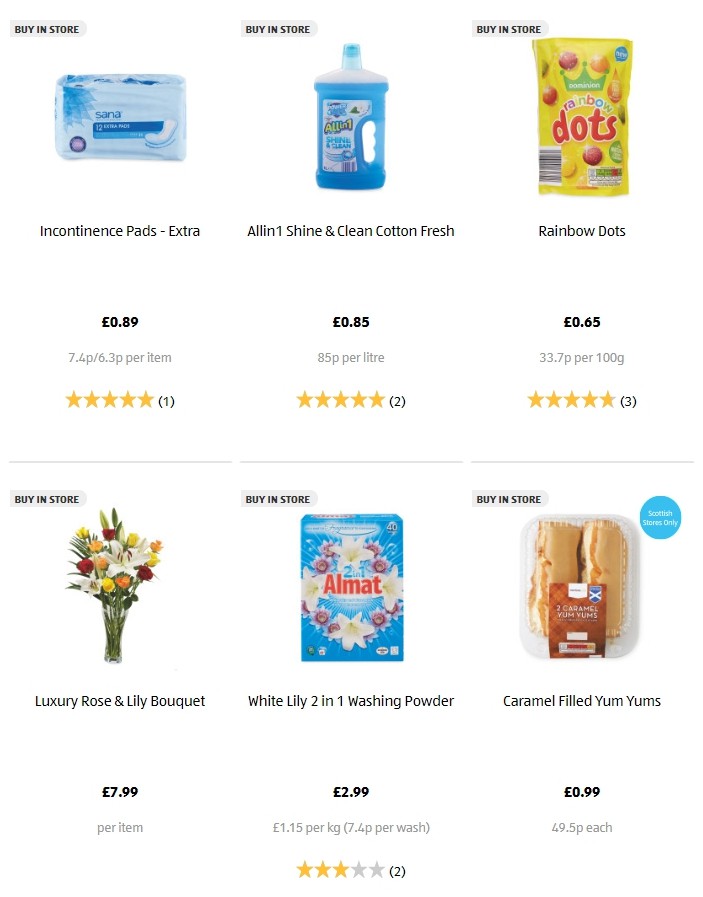The color screenshot depicts a shopping page on a market website featuring six different home goods items against a white background. Each item has a "Buy in Store" button above it that is currently grayed out. The detailed breakdown of the items is as follows:

1. **Incontinence Pads (Extra Size)**:
   - Displayed price in pounds.
   - Smaller text indicating the price per item.
   - A review section showing that one person has reviewed the product.

2. **All-in-One Shine and Clean Cotton Fresh Cleaning Liquid**:
   - Displayed price in pounds and price per liter.
   - A star rating indicating customer reviews.

3. **Rainbow Dots Candy**:
   - Packaged in a yellow wrapper with an illustration of candy dots.
   - Displayed price in pounds and price per item.

4. **Bouquet of Flowers**:
   - No additional details visible in the screenshot.

5. **Washing Powder**:
   - Displayed price in pounds and price per kilogram.
   - A star rating with three out of five stars.

6. **Pastry**:
   - No additional details visible in the screenshot.

The layout is structured with three items on the top row—Incontinence Pads, Cleaning Liquid, and Rainbow Dots Candy—and three items on the bottom row—Bouquet of Flowers, Washing Powder, and Pastry. The Washing Powder is distinct in having a visible star rating.